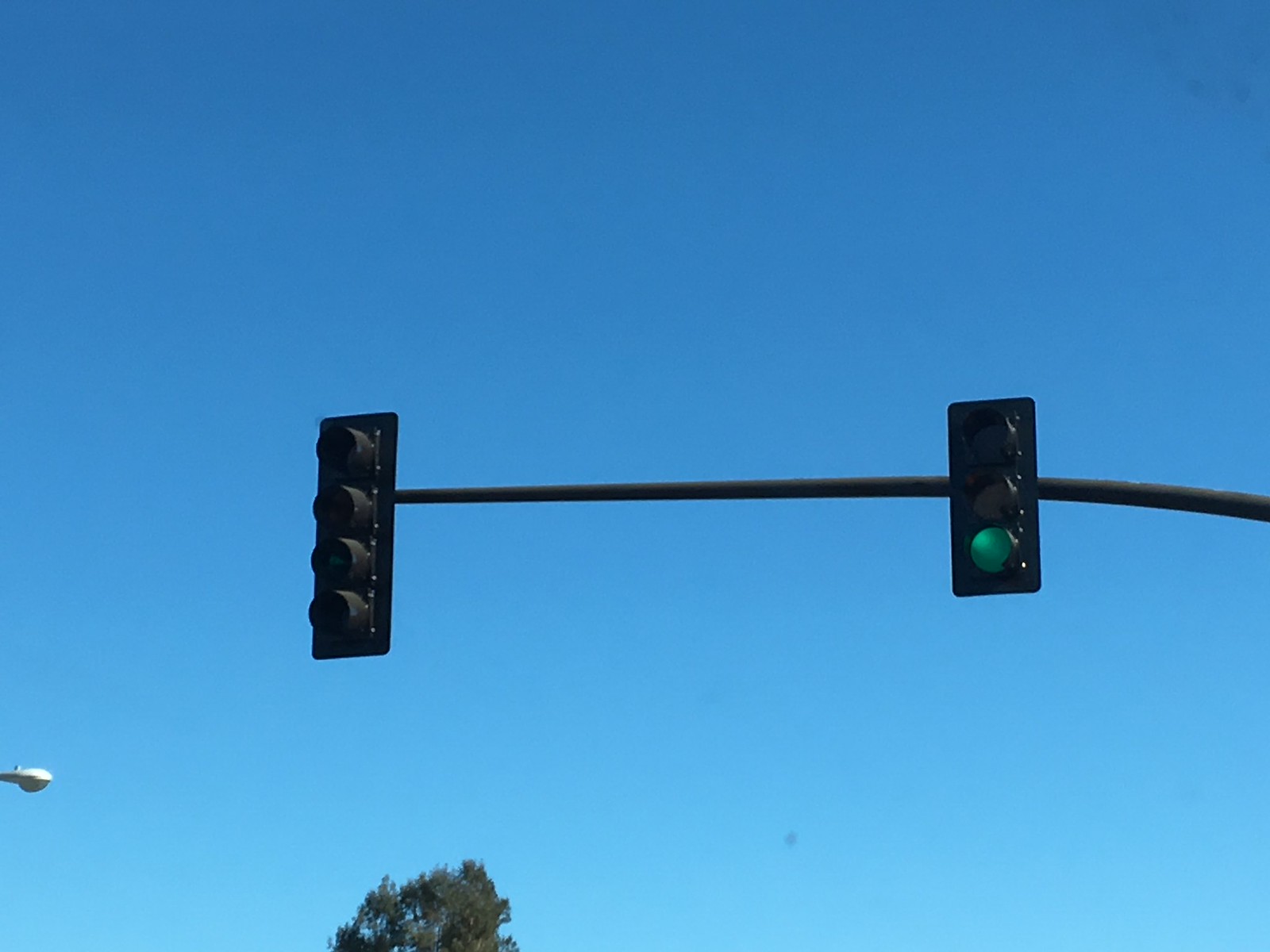The image, taken at a stoplight on a clear, sunny day, features a beautiful blue, cloudless sky that dominates the background. Toward the bottom left-hand corner, the top of a pine tree and the bulb of a streetlight can be seen. Stretching horizontally from the middle right-hand side of the image to about the left third is a black pole. Attached to this pole are two black traffic lights. The traffic light on the right has three bulbs, with the green light currently lit, indicating cars in that lane can proceed. On the left, a separate traffic light with four bulbs hangs farther out into the intersection but is currently not lit. The entire setup creates a striking contrast against the serene blue sky.